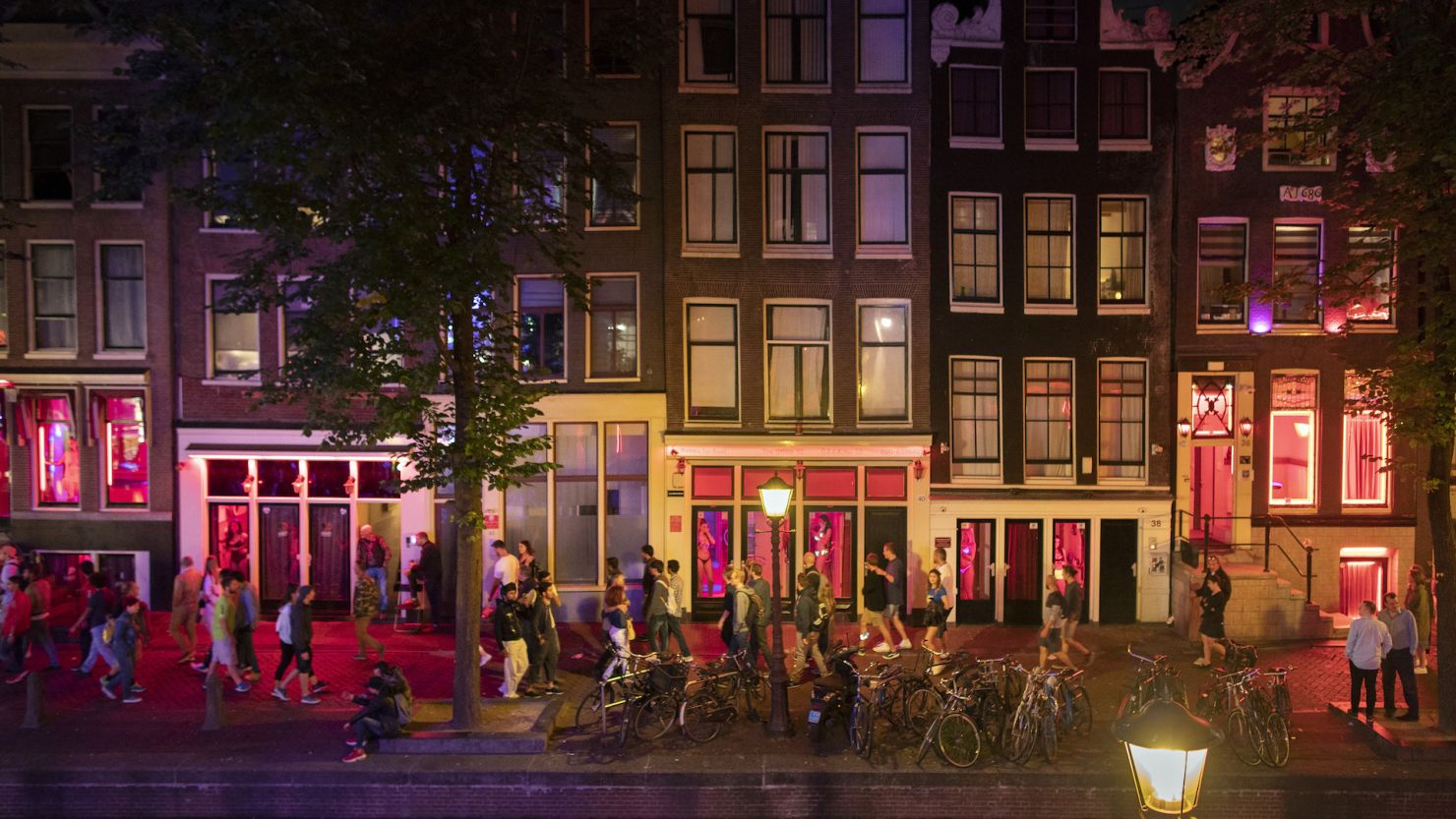This color photograph captures a vibrant urban street at night. The scene opens with a curved street at the very edge of the foreground, leading up to a bustling brick-paved sidewalk. To the right, bike racks brimming with bicycles line the walkway, hinting at the area's popularity among cyclists. Two trees, their bases encased in stone walls, stand prominently. Perched on one of these walls, to the left, are two people engaged in conversation.

The sidewalk is alive with pedestrians strolling in various directions, adding a dynamic essence to the setting. Behind the walkway, an array of multi-story buildings unfolds. The architecture predominantly features red-brick exteriors with windows framed in white, some of which are illuminated, casting a warm glow onto the street.

Among the storefronts, some display images of women in bikinis, suggestive of Amsterdam’s nightlife and its renowned Red Light District. The scene is a mosaic of urban life, seamlessly blending historical architecture with contemporary city living.